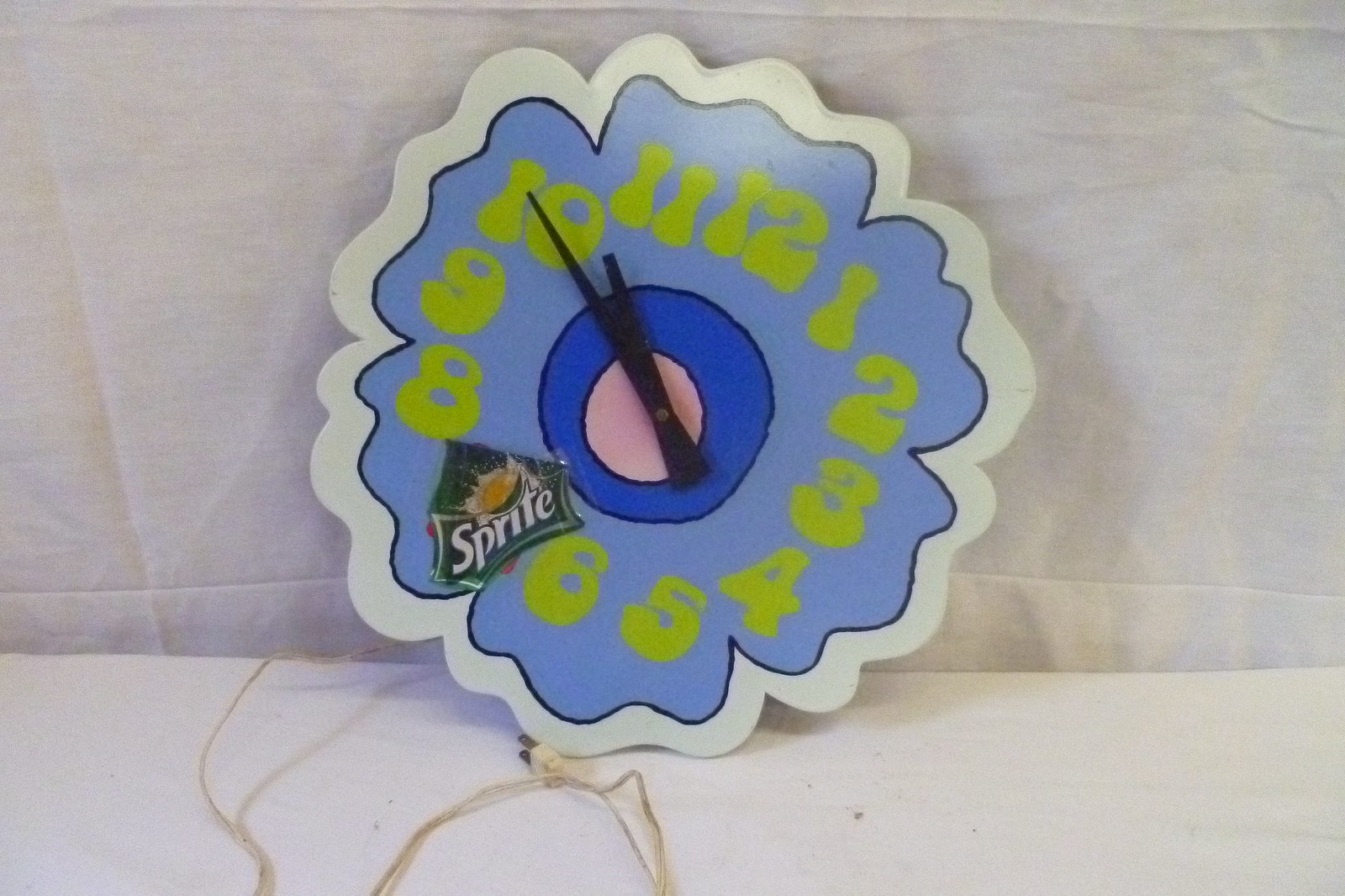This photograph features a uniquely crafted wall clock designed to resemble a vibrant blue flower with six wavy petals. The clock, which appears to be made from cardboard or paper, rests on a white shelf against a gray wall. Its design suggests a child’s artistic touch, emphasized by its rough, whimsical contours. The clock face is adorned with bright green, blocky numbers that have a cartoonish flair. Notably, where the number 7 should be, there is a prominent Sprite advertisement sticker, superimposed over an original flower sticker. The clock’s center showcases concentric circles—a dark blue one followed by a pink or flesh-colored one. Black hour and minute hands mark the time, and a transparent cord with a white plug is visibly draped around the bottom, adding to its quirky charm.